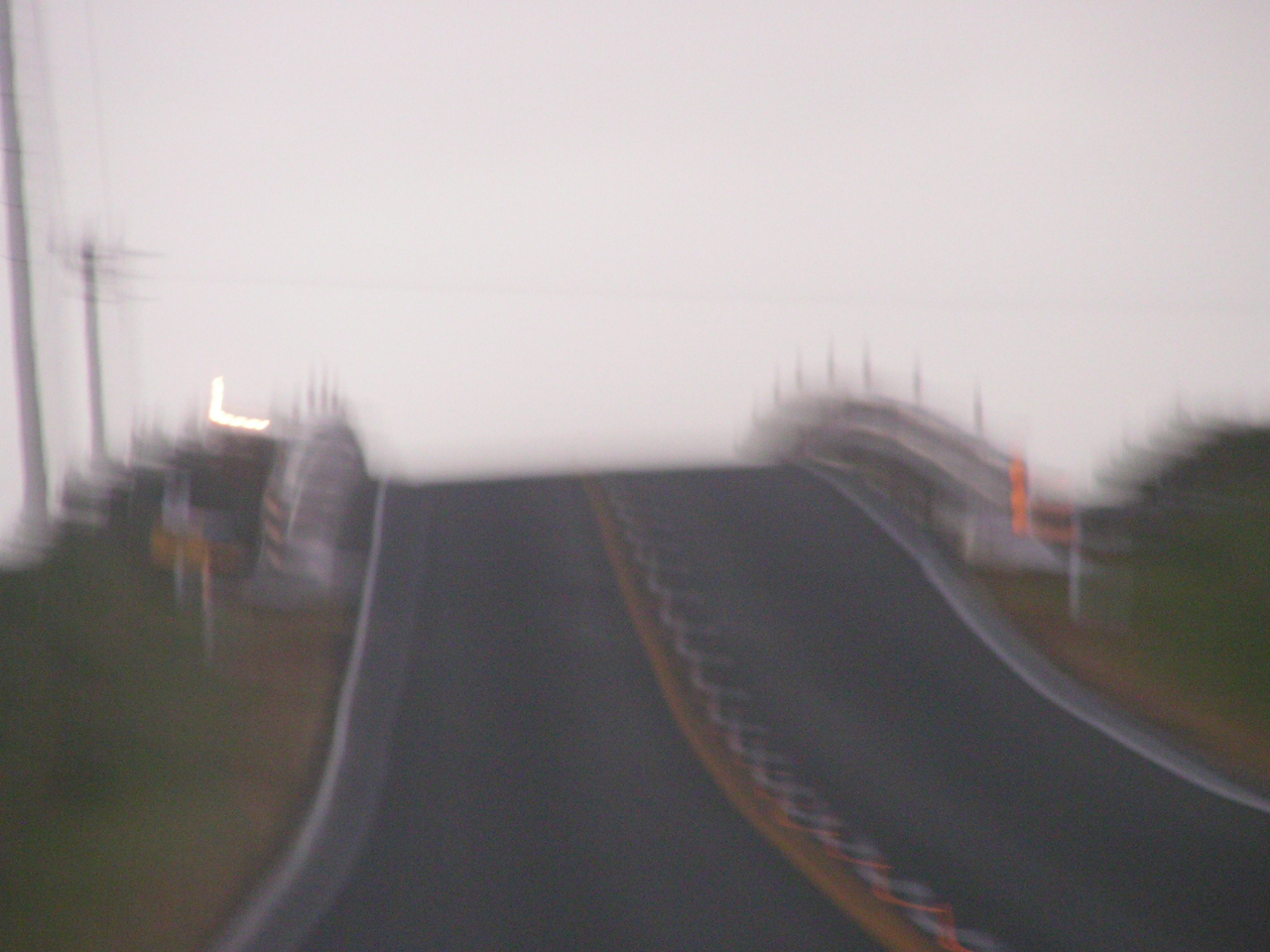A blurry photo taken at twilight depicts a black asphalt two-lane road ascending a hill, likely connecting to a bridge. The road, marked with a double yellow line on the left and a dashed white line on the right, indicates a two-way passage. Metal barricades with orange reflectors line the ridge, accompanied by warning signs signaling caution. Strips of verdant and dead grass appear along the shoulders of the road, which is flanked by either another road or bushes. The overcast sky casts a gray blanket over the scene, muted by low light conditions. On the left side, two metal poles with power lines stretch from top to bottom, with an additional power line crossing the entire width of the image.